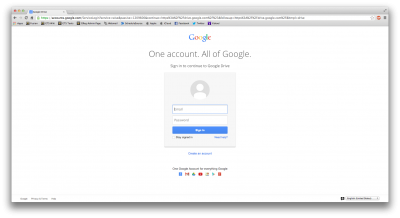A screenshot depicting the main Google sign-in page. The image shows Google's familiar multi-colored logo at the top, accompanied by the text "One account. All of Google." Centered on a plain white background, the login section features fields for entering an email and password, with a sign-in button below them. To the right of these fields, a grayed-out user icon is visible. Below the sign-in area, there are indiscernible small texts, possibly explaining additional features or options. Various Google service icons, such as Gmail and YouTube, are noticeably present, hinting at the functionalities accessible through a Google account. The screenshot appears to have been captured within a Chrome browser, evidenced by the metallic-tinted border and the red, yellow, and green stoplight buttons in the upper left corner, typical of a Chrome window. The upper section of the image also shows multiple tabs open, although their details are not discernible.